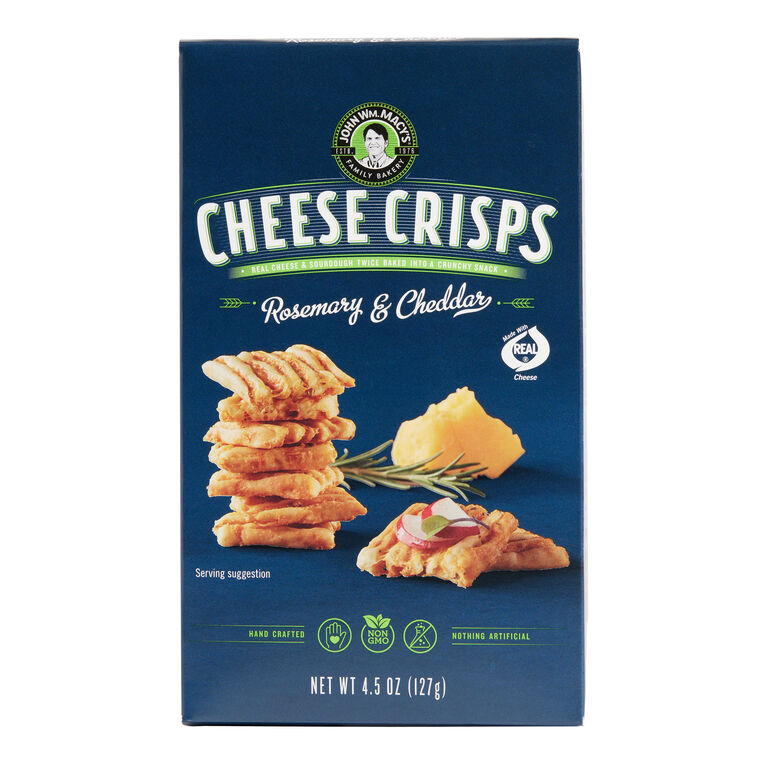This photograph displays a box of John W. M. Macy's Cheese Crisps in blue packaging, set against a solid white background. The box features a deep blue hue at the top, transitioning to a light blue at the bottom. At the upper section of the box, a light green circular logo showcases a black-ink drawing of a person's face, with "John W. M. Macy's" and "Family Bakery" written in arcs around it. Below the logo, the words "Cheese Crisps" stand out in large white letters, bordered by thin horizontal light green lines, and a thicker green band beneath them with illegible white text. Further down, "Rosemary and Cheddar" is prominently displayed. The front of the box includes a visual representation of the cheese crisps piled up, resembling puffed-up snacks similar to pork rinds. Additionally, a single crisp is depicted with a red substance, a leaf, and a small slice of cheese, possibly white cheddar. The net weight of the package is labeled as four and a half ounces.